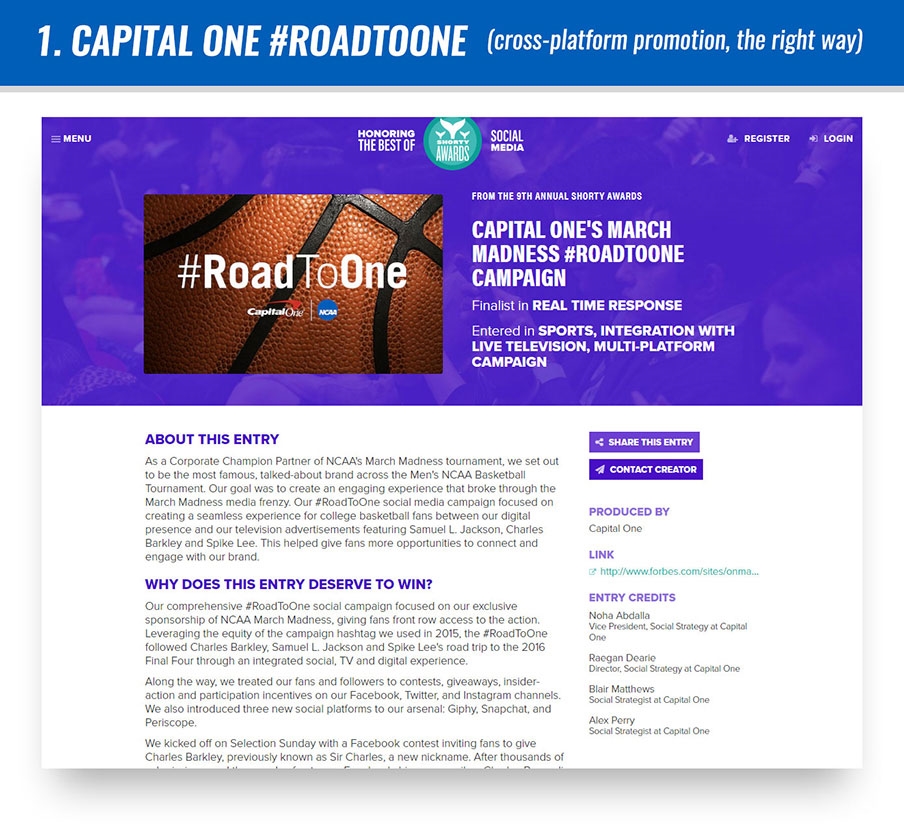The image features a website with a bold blue background and large white text proclaiming "Number One Capital One #RoadToOne." A prominent purple box overlays the design, containing a close-up image of a basketball's textured surface. The text in the box reads "#RoadToOne" with "Capital One" underneath it.

In the upper left-hand corner, there is a menu bar. This entry is presented as a finalist in the Real-Time Response category at the 9th Annual Shorty Awards. The campaign, titled "Capital One's March Madness #RoadToOne Campaign," is highlighted under the Sports Integration with Live Television Multi-Platform Campaign section.

The website details the "About This Entry" section, explaining that the goal was to create an engaging experience that stood out amidst the March Madness media frenzy. The "Why Does This Entry Deserve to Win" section elaborates on Capital One's exclusive sponsorship of March Madness, emphasizing how they provided fans with front-row access to the action. Throughout the campaign, they engaged fans and followers with contests, giveaways, interaction, and participation incentives across Facebook, Twitter, and Instagram platforms.

Additionally, the page includes options to share the entry and contact the creator, with a link and acknowledgment that the campaign was produced by Capital One.